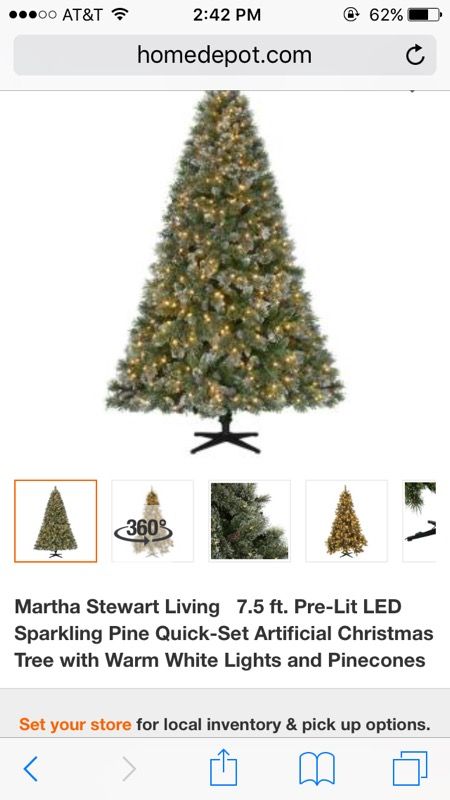A screenshot from a smartphone with AT&T service, showing a full signal and a 62% battery at 2:42 p.m., captures a webpage from homedepot.com. Featured prominently in the image is a Christmas tree listing: the "Martha Stewart Living 7 1/2 ft. Pre-Lit LED Sparkling Pine Quick-Set Artificial Christmas Tree with Warm White Lights and Pine Cones." The tree is beautifully decorated and is showcased from various angles below the main image, highlighting its warm white lights and the addition of pine cones—a nice touch in its design. The webpage also includes an option to "Set Your Store," prominently displayed in orange, to check local inventory and pickup options. Navigation icons, such as an arrow to the left, a page up, a book icon, and overlapping pages, are situated across the screen.